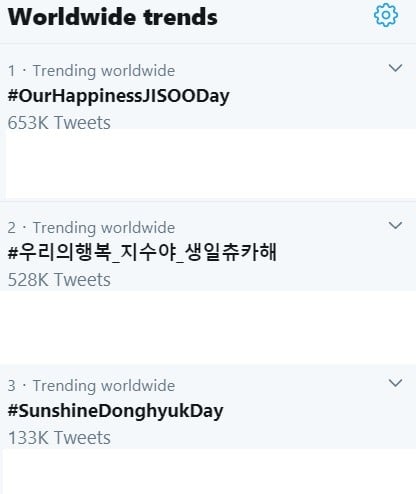The image is a vertical list featuring alternating light blue ribbons and white spaces. It showcases worldwide trending topics. At the top, the first light blue ribbon displays "Worldwide Trends" in black text with a blue settings icon on the far right. Below, the first trend is marked as "1. Trending Worldwide," featuring the hashtag "#OurHappinessJISOOday," which has amassed 653,000 tweets.

The following white space separates the next light blue ribbon, labeled "2. Trending Worldwide," presenting text in either Japanese or Chinese characters, and it indicates 528,000 tweets.

Another white space precedes the final light blue ribbon, labeled "3. Trending Worldwide," highlighting "SunshineDonghyukDay," precisely spelled "Sunshine D-O-N-G-H-Y-U-K Day," which has garnered 133,000 tweets.

Each light blue ribbon includes an arrow icon, suggesting that the sections are expandable for additional details.